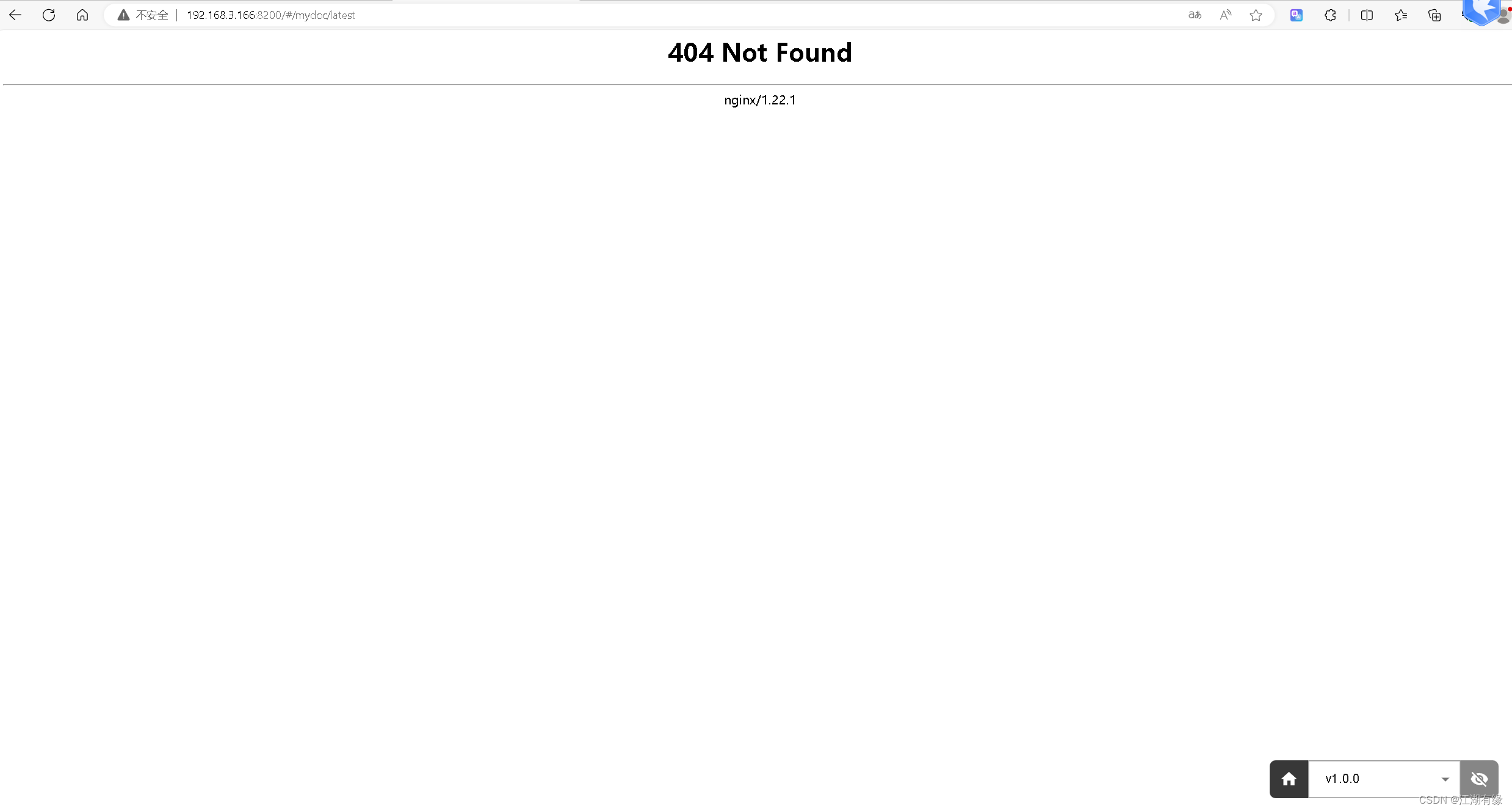A screenshot captures a seemingly web-based page displaying a "404 Not Found" error in large, bold black letters prominently centered on the page. The URL of the page, positioned just above the error message, is too minuscule to decipher. Below the "404 Not Found" message, there appears to be an error return code, although the text is unfortunately too small to read. The overall layout is typical of a web error page, indicating that the requested resource could not be found.